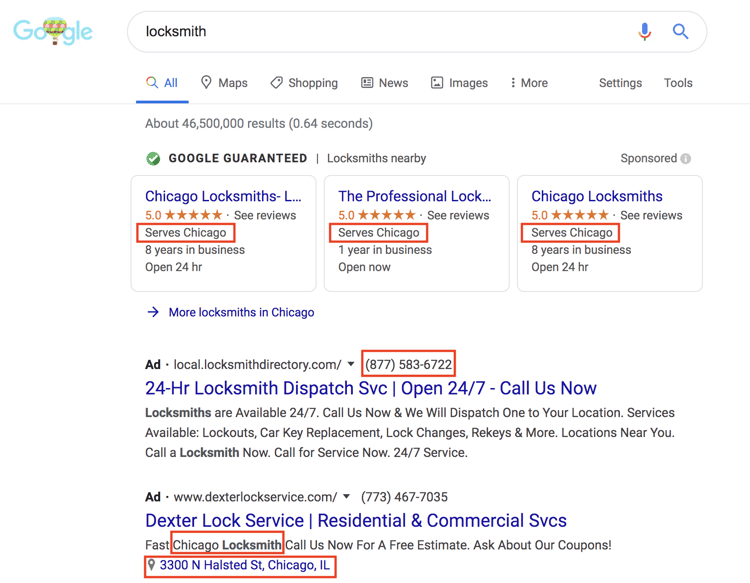This screenshot captures a Google search results page specifically for the query "Google Guaranteed Locksmiths Chicago." It illustrates a unique advertising format employed by Google. Notably, five locksmith services are prominently featured, with the top three results labeled as "Google Guaranteed." Each listing includes a phone number wrapped in red boxes for emphasis.

Additionally, the search indicates that Google returned approximately 46 million results in just 0.64 seconds. The familiar Google interface elements, such as "All," "Maps," "Shopping," "News," "Images," "More," "Settings," and "Tools" are present beneath the blue "Google" logo. Interestingly, the "Google" logo appears to have a parachute integrated into its design, adding a unique visual twist.

Moreover, the screenshot highlights "Dexter Lock Service" and other locksmith services in Chicago. A red ribbon can be seen accentuating certain parts of the search results, and two advertisements appear below the guaranteed listings.

Overall, the image showcases how Google provides a blend of organic, guaranteed, and paid listings for users searching for locksmith services in the Chicago area.